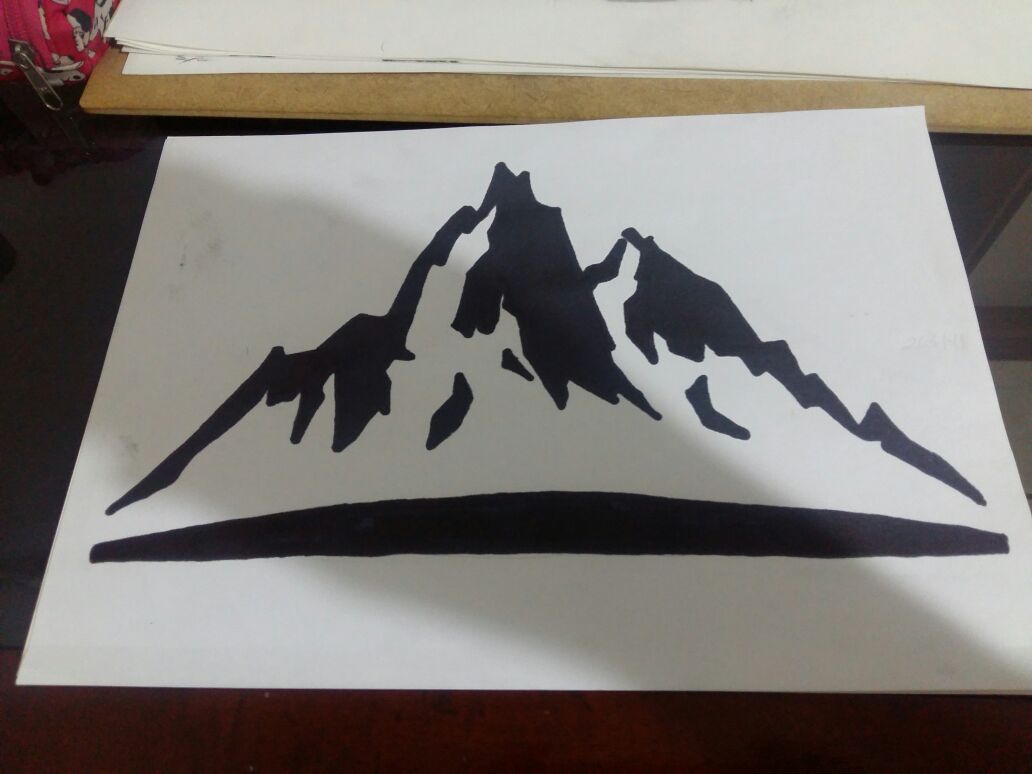This image, created on a white sheet of paper, depicts a striking mountain landscape. The mountains are depicted in contrasting shades of black and white, suggesting a natural dusting of snow on their peaks. The artist skillfully uses the white areas to represent snow accumulations in the crevices of the mountains, creating a realistic and expressive portrayal of a wintry scene.

Towards the lower portion of the image, an oval-shaped black formation adds depth, contributing to a three-dimensional effect. The background is also white but marred with black smudges, likely the result of charcoal or crayon work, adding a raw and textured element to the artwork.

This paper rests on a sleek black desk that features a maroon border at the front, adding a touch of elegance to the display. Behind the desk, there is a red bag and a board, providing context to the setting and grounding the scene in a real, lived-in space.